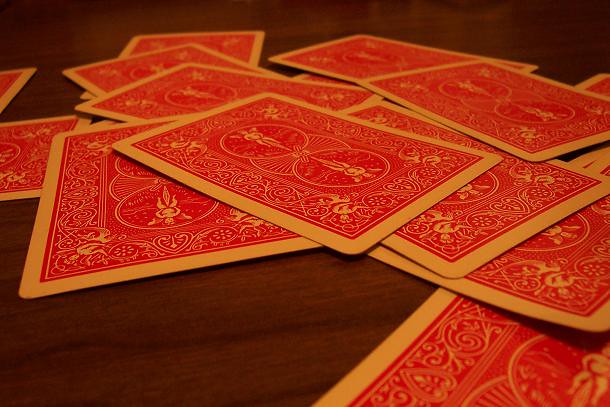The image presents a zoomed-in view of a wooden surface, likely a table, taken from an angle with the lens positioned on the left side. The table's surface is rich brown with darker grain lines running through it. The detailed texture of the wood is noticeable in the bottom left corner and the top of the image, offering an almost tactile perception of its rugged and natural finish.

Scattered across the table are playing cards, predominantly gathered from the upper left-hand side down to the bottom right. The cards are facedown, displaying their red backs adorned with white borders. In the center of these red backs is a distinct pattern mimicking a Venn diagram—three overlapping circles. The central circle features white and red stripes, while the two flanking circles on either side contain small white figures, although details blur upon closer inspection.

The arrangement of the cards lacks order; they lie in a casual, haphazard manner. Some cards pile messily in the center while others rest individually, particularly noticeable on the left-hand side. A portion of the cards extends beyond the frame, particularly at the bottom, cutting off the view of a complete layout but highlighting the informal spread of the deck.